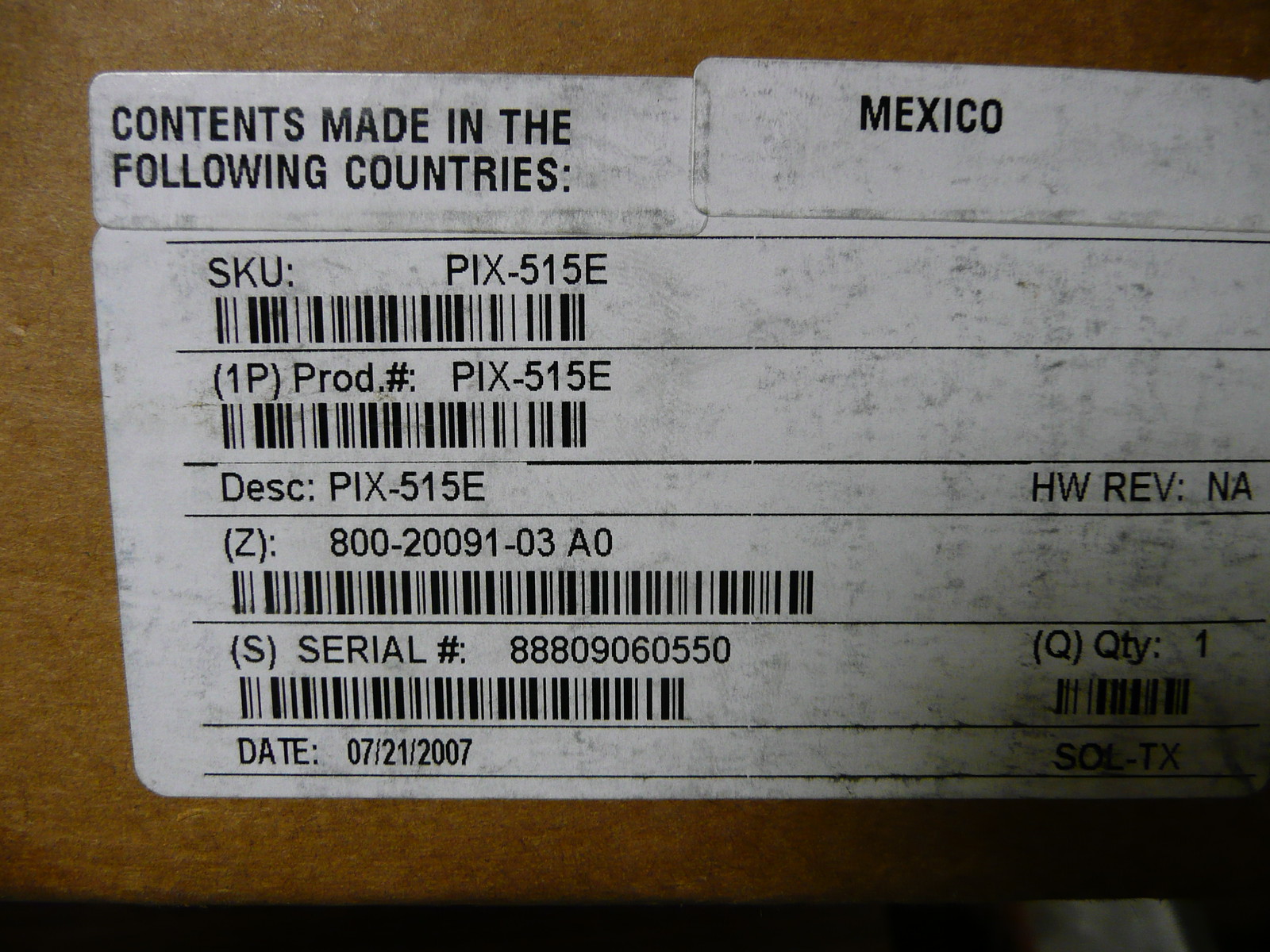The image features a close-up of a light brown cardboard box with a detailed white label on its side. The label is rectangular with curved edges and is densely printed with black ink. At the top left corner of the label, it reads "CONTENTS MADE IN THE FOLLOWING COUNTRIES" followed by "MEXICO" in capital letters. Below this, the label is segmented into several sections with multiple lines of text and barcodes. The first barcode is labeled "SKU: PIX-515E", followed by another barcode with "Prod Number: PIX-515E". Further down, there's another barcode labeled "Description: PIX-515E" with the code "Z: 800-20091-03 A-0". Below this, there is the "Serial Number: 888-090-60-550" next to another barcode. Finally, the label displays the date "07/21/2007," which likely indicates a production date. Additionally, on the right side, it says "HW REV: NA" followed by "QTY: 1". This descriptive label organizes a wealth of product information including manufacturing details, identification codes, and logistical data.